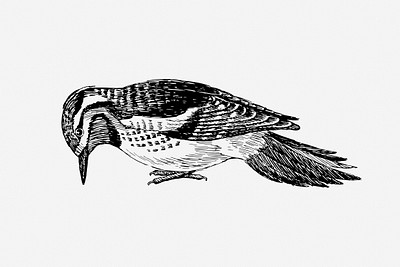This detailed black and white sketch depicts a woodpecker in a horizontal orientation on a blank white background. The medium-sized bird is centrally positioned on the paper, portrayed standing on its two legs, as if ready to peck at something on the ground. The sketch clearly shows the bird's characteristic posture with its beak facing downward.

The woodpecker's plumage is meticulously detailed, emphasizing the different textures and sections of its feathers on its tail and wings. The upper part of the tail is white, transitioning to black feathers towards the tip. The top of the bird's body is predominantly black with a few white patches, including a distinctive white stripe on its face.

The bird's breast and belly areas are mostly white, contrasting with its darker upper parts. Its feet, illustrated in black or gray, display defined nails. The left side of the woodpecker, facing the viewer, reveals a single beady eye rendered in a way that gives it a shiny appearance, adding a touch of liveliness to the depiction. Overall, the drawing is highly detailed, showcasing various shades of gray to highlight the bird's natural coloring, and it conveys the woodpecker's typical behavior of searching for food.